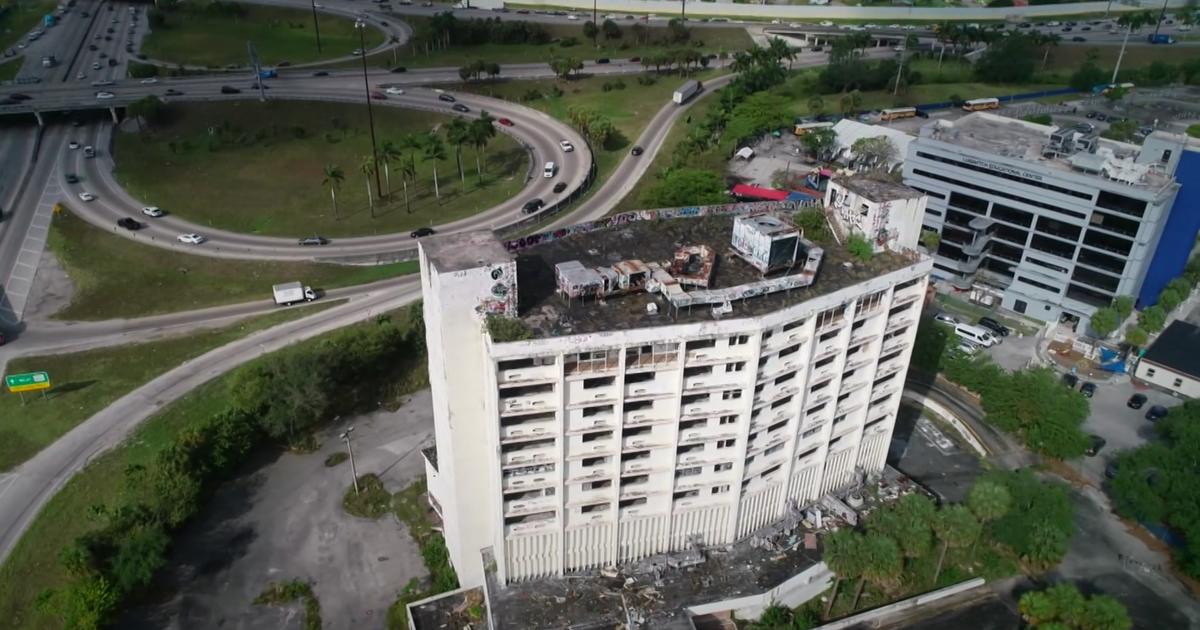This aerial photograph captures a detailed urban scene centered around a tall, white building, possibly a condemned or under-demolition apartment structure. The building is at least seven to eight stories high and topped with extensive AC equipment. Surrounding the building are green lawns and a variety of trees, including some palm trees, contributing to a tropical ambiance reminiscent of areas like Florida. Adjacent to the white building is a tall, gray structure that appears to be a parking garage, with a few cars parked in front of it.

In the distance, the complex network of highways and overpasses full of vehicles can be seen, including a distinct roundabout exit. This background also features numerous looping roads intersecting the urban landscape. Amidst the trees, tall lights stand visible, adding to the city's infrastructure. There is mention of some debris and an old, possibly run-down parking lot, underlining the juxtaposition of developed and deteriorating elements within the same vicinity. The tropical setting, combined with the mixture of thriving and decrepit structures, imparts a sense of both vibrancy and decay within the cityscape.